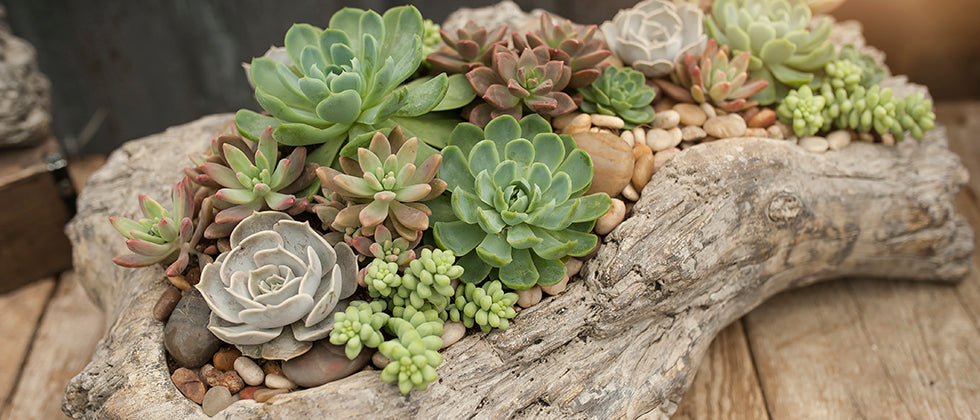The photograph depicts a hollowed-out tree trunk that contains an arrangement of various succulents and stones. The tree trunk, with its light brown to dark grayish hue, serves as a natural planter for the succulents, which range in color from light gray and off-white green to dark green with some even featuring dark red edges. The succulent varieties also differ in size and shape, with some bearing small, grape-like leaves, while others have larger, flower-like formations. This intriguing setup is placed on a wooden surface made of vertically aligned two-by-fours. In the lower left-hand corner of the photo, there is a small wooden box with an unidentified object on top. The entire scene exudes a rustic charm, merging natural elements with artistry.